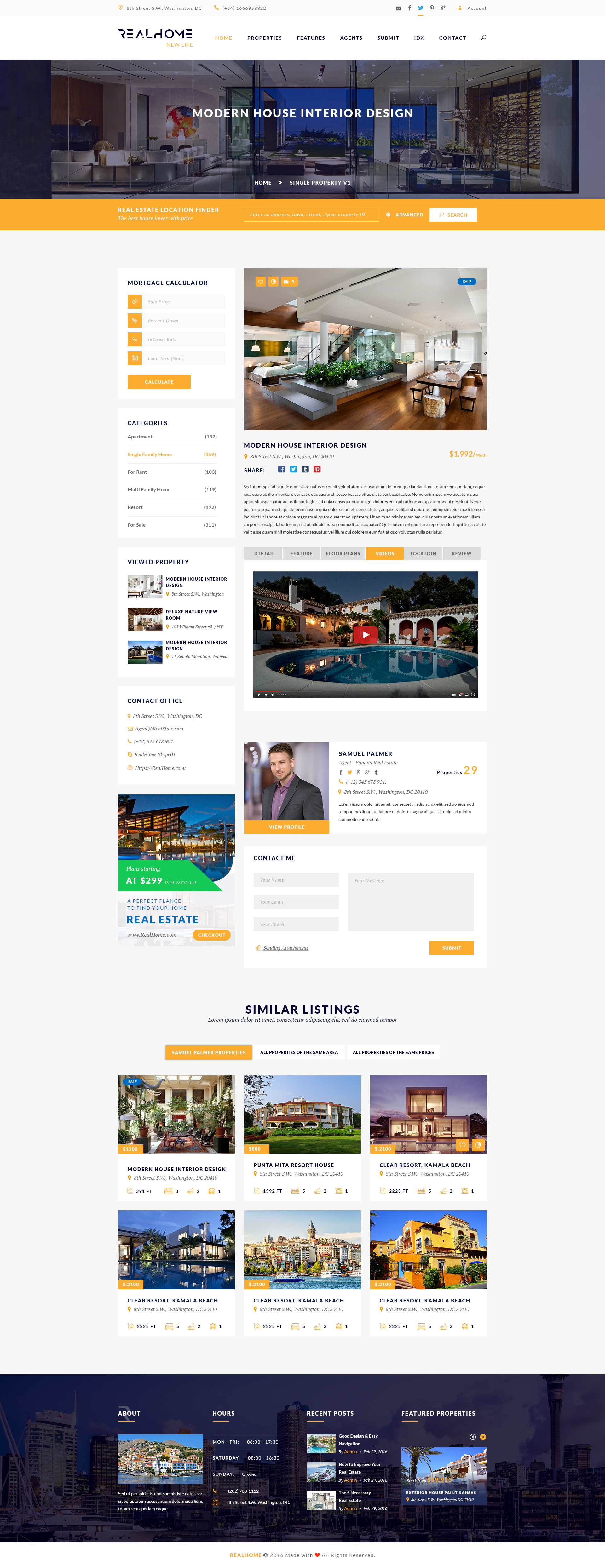This image features a detailed layout of a web page dedicated to showcasing modern house interior design. At the top, there is a white taskbar with the legible text "Real Home Logo." Below that, there's a large banner with an image depicting the inside of a room, showcasing white walls, a view through a window, and some blue hues in the background. The banner prominently displays the text "Modern House Interior Design" in white, which stands out as the largest lettering on the page. Under this banner is an orange taskbar, and to the left, there appears to be some kind of poll represented by orange graphics. 

On the right-hand side of the banner, a detailed photo shows a room with a wooden floor, a white ceiling, green foliage, and a long white dining table. The green plants are situated on a central platform. Further down, text and orange boxes populate the layout, including a visible YouTube video thumbnail featuring a blue swimming pool, a white building, and surrounding greenery. Beside the pool image is a man wearing a purple shirt and suit jacket, with another house in green and blue tones shown to the bottom left of him. The bottom section of the image showcases a row of six house images, followed by a dark purple banner at the very bottom, containing small outdoor-themed images. Each segment is carefully placed, creating a visually engaging and informative display that guides viewer attention through various elements of modern home design.